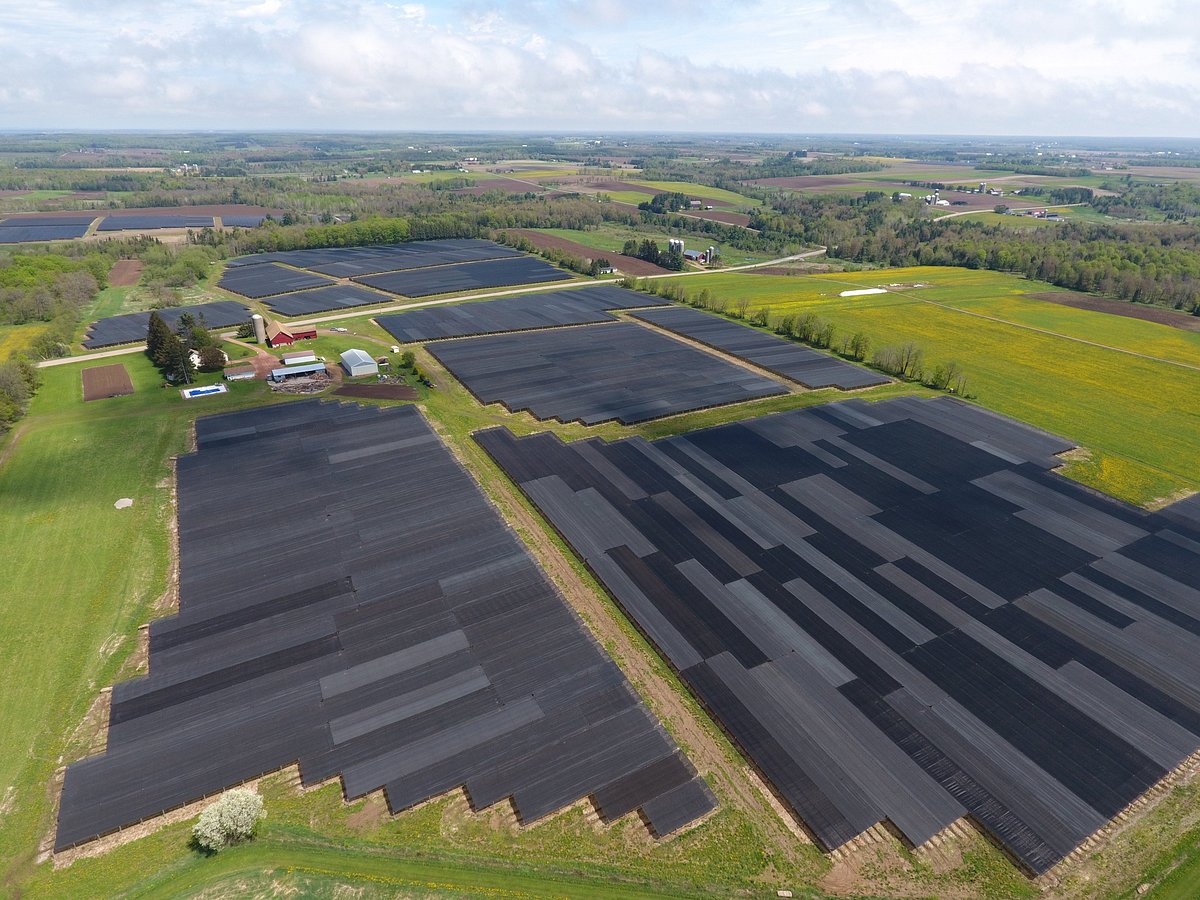This aerial photograph, likely taken by a drone, showcases a sprawling farmland with various features. Dominating the image are verdant green fields interspersed with nine distinct patches of black and gray panels, each rectangular and varied in shade, creating a geometric pattern. At the top middle left of the image, a farmstead is visible, consisting of a house, possibly a barn, and several storage buildings. More greenery stretches out into the distance, dotted with smaller structures that may be additional houses. The sky above is a light blue, adorned with scattered white clouds, contributing to the serene rural atmosphere. The image captures a bird's-eye view of a vibrant agricultural area set against the backdrop of a picturesque countryside.